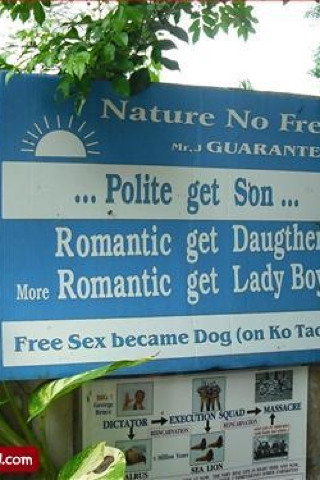The image depicts a perplexing outdoor sign framed by tree branches and leaves at both the top and bottom, with a clear sky visible in the background. The sign itself is blue with white text, featuring a Sun symbol at the top. The readable portions of the text include fragmented and confusing phrases, starting with "nature no" and "FRE," followed by "Mr. Guarantee," although parts of these sections are cut off. Beneath that, a white banner with blue font declares "polite get son... romantic get daughter... more romantic get ladyboy." Another white banner reads, "free sex became dog on co tat," but this too is incomplete. Additionally, there's a small, difficult-to-decipher picture below this text, possibly featuring the word "dictator" with arrows pointing to words like "execution squad" and "massacre." The overall content of the sign is chaotic and unclear, seemingly mixing humorous elements with stark, inappropriate messages, leaving its purpose ambiguous and confusing.